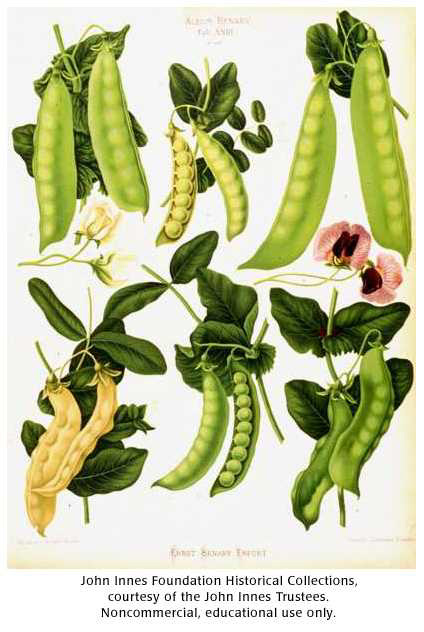This vertical illustration features six detailed images of various pea pods, some of which are green while others exhibit a yellow hue. Each pea pod is attached to its stem and adorned with leaves, showing different stages of maturation. Some pods are closed with visible peas beneath the thin covering, while others are partially open, revealing rows of peas inside.

The pods are arranged in two rows. In the upper row, the first illustration shows a pair of pods with yellow peas visible through the semi-transparent green shell. The second shows a smaller pod with the covering peeled away to reveal yellow peas, all set against a backdrop of green leaves. The third depicts long, slender, light-green pods.

In the bottom row, the first set of pods are yellow, with bulbous sections hinting at the peas inside, framed by green leaves. The middle image also has two pods; one closed and light green, the other peeled back to reveal a dozen green peas within, surrounded by foliage. The final set shows two small, bent pods with the outline of peas visible through the shell, again accompanied by leaves.

Completing the illustration are small flowers, with a yellow bloom in the upper left and rose-pink flowers in the lower right. The text, describing the illustration as part of the "John Innes Foundation Historical Collections, courtesy of the John Innes Trustees, non-commercial educational use only," is set against a white background in a sans-serif font.